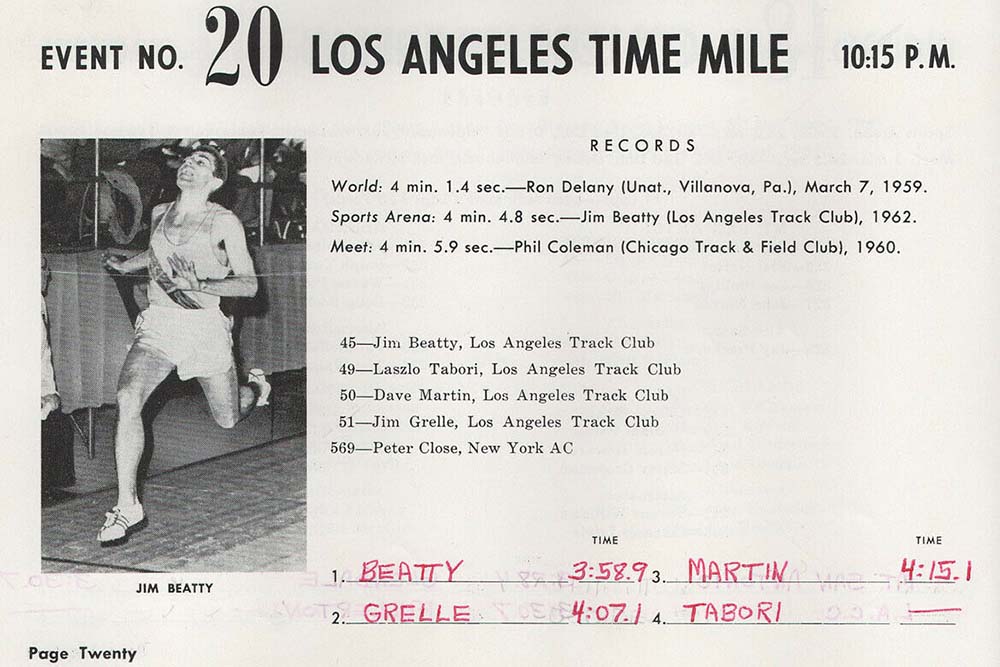This detailed image appears to be a scan of a printed event record card, capturing the historical achievements in a track and field event. At the top, it prominently features the black text: "Event Number 20, Los Angeles Time Mile, 10:15 PM." The central visual element is a black and white photograph of an athlete, Jim Beatty, running while wearing a sleeveless shirt and shorts. His name is labeled beneath his picture as "Jim Beatty, B-E-A-T-T-Y." 

To the right of the photograph, there is a list under the heading "Records." This section records significant time milestones:
- "World" record: 4 minutes 1.4 seconds, set by Ron Delaney, Unattached, Villanova, Pennsylvania, March 7, 1959.
- "Sports Arena" record: 4 minutes 4.8 seconds, achieved by Jim Beatty of the Los Angeles Track Club in 1962.
- "Meet" record: 4 minutes 5.9 seconds, established by Phil Coleman from the Chicago Track and Field Club in 1960.

Below this list, additional black text delineates participant numbers and names:
- 45: Jim Beatty, Los Angeles Track Club
- 49: Laszlo Tabori, Los Angeles Track Club
- 50: Dave Martin, Los Angeles Track Club
- 51: Jim Grell, Los Angeles Track Club
- 569: Peter Close, New York A.C.

Handwritten in red text on lined sections are the recorded times for the event:
1. Beatty: 3 minutes 58.9 seconds
2. Grell: 4 minutes 7.1 seconds
3. Martin: 4 minutes 15.1 seconds
4. Tabori: no time recorded (indicated by a crossed-out line)

The format suggests this card was used to officially log and recognize timing records during a track meet, providing a meticulous account of performance metrics and athlete details.